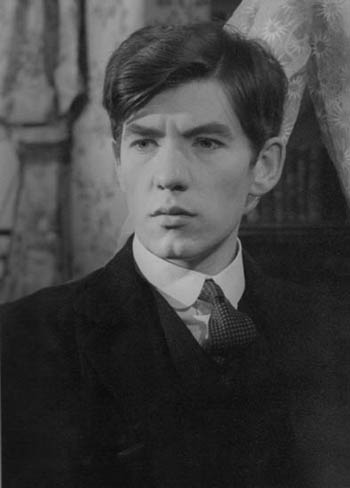A striking black and white photograph captures a young Caucasian man, likely in his mid-20s, donning a formal attire. He wears a black jacket paired with a matching black vest, complemented by a dark tie adorned with rows of white dots. His crisp white shirt features a notably stiff collar. His medium-length hair, styled above the ears with long bangs at the front, enhances his serious air. His expression is intense and somewhat menacing; his gaze, directed off-camera towards the front left of the viewer, is framed by slightly raised eyebrows. A pronounced dimple is visible on his chin, adding character to his stern visage. The backdrop includes lacy, curtain-like material and a glimpse of a wall. To the right behind his head, dark images of books on a shelf suggest an intellectual setting. The overall aesthetic and his hairstyle evoke a 1960s vibe, making the photo reminiscent of a still from a black and white movie from that era.